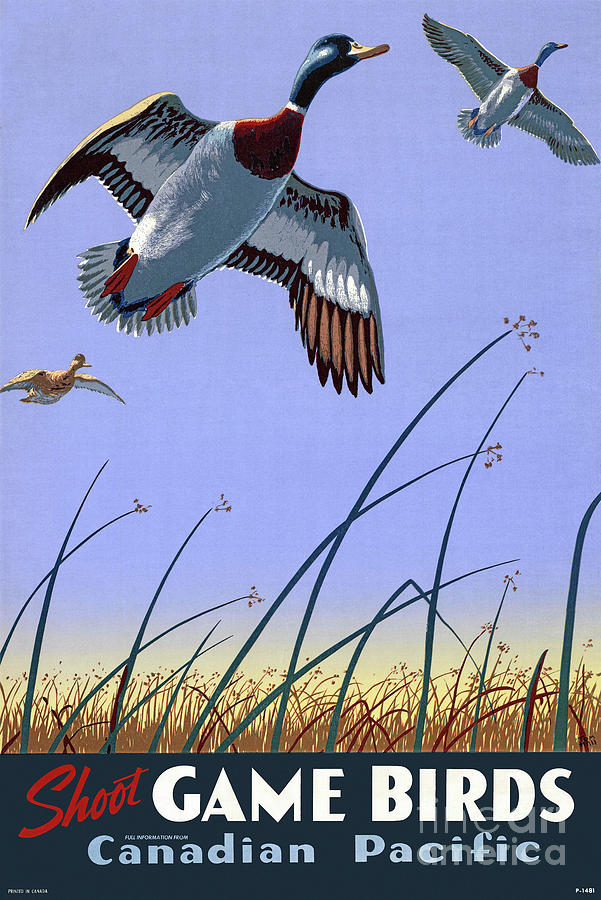This is a detailed poster promoting "Shoot Game Birds" by Canadian Pacific. The image showcases three vibrant game birds, likely mallards, in mid-flight against a soft, light blue sky with hints of sunlight on the horizon. The birds are beautifully detailed, featuring rich colors: two have striking green heads, brown necks, and white bodies, while the third, slightly different species in the background, is adorned in brown and white. They glide not far above a field of tall, brown and green grasses, adding a sense of natural motion to the scene. The perspective is from a low angle, creating an upward-looking view towards the serene sky. At the bottom of the poster, the text "Shoot Game Birds" stands out with "shoot" in red, "game birds" in white, and "Canadian Pacific" in light blue, grounding the drawing with its promotional message. The overall composition harmonizes vivid wildlife details with a tranquil, earthy landscape, evocatively capturing the essence of game bird hunting.